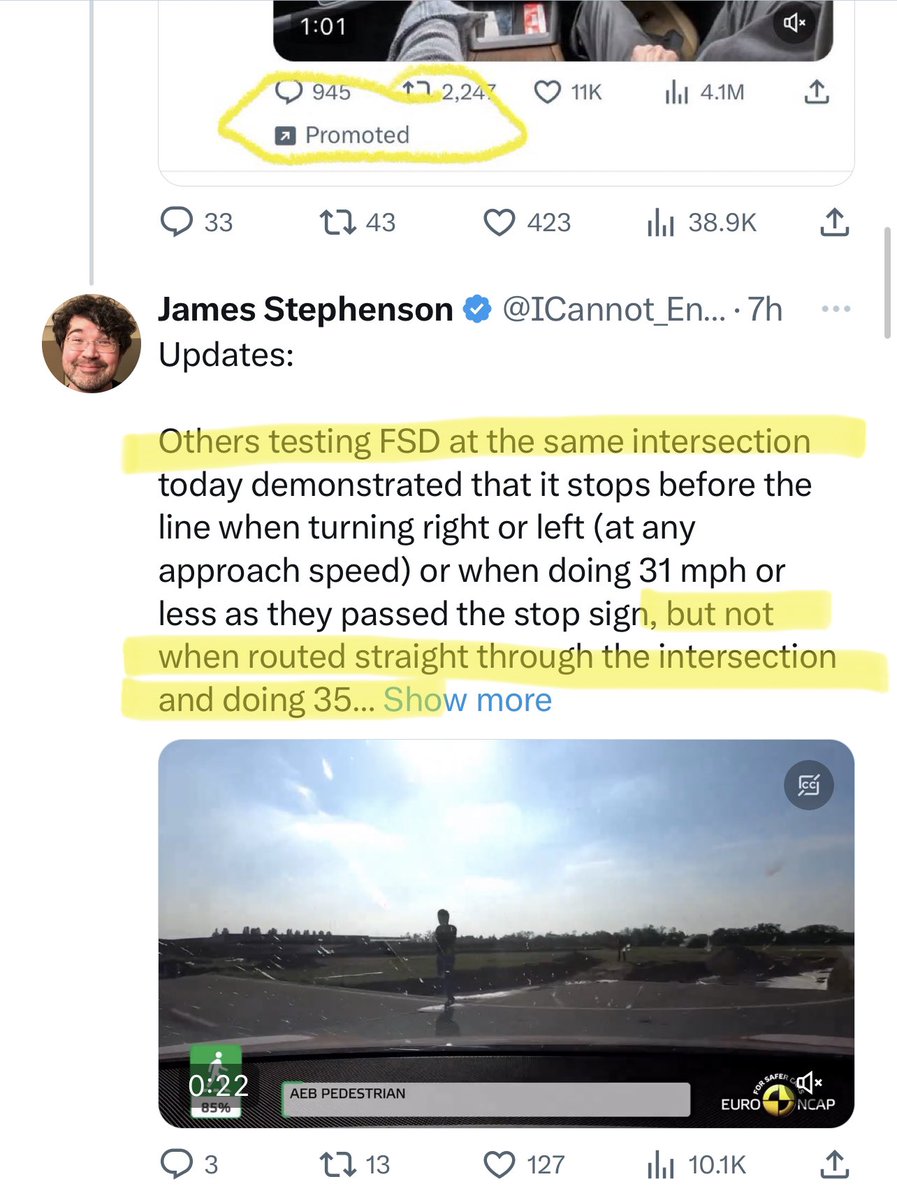**Detailed Caption:**

The screenshot appears to be from Twitter, based on the layout and design. The top section of the image contains the bottom part of a video post, which seems cropped and shows "101" views and a muted volume icon. Below that, the main tweet is highlighted, with interaction metrics including 945 comments, 2,247 retweets, 11,000 likes, and 4.1 million views. The word "Promoted" is circled in yellow in a haphazard manner, likely done using a screen drawing tool.

A reply from James Stevenson, identifiable by his verified checkmark and partial username "@I cannot underscore EN…" posted seven hours earlier, is highlighted. In his reply, the text "Others testing FST at the same intersection today demonstrated that it stops before the line when turning right or left at any approach speed, or when doing 31 miles per hour or less as they pass the stop sign, but not when routed straight through the intersection and doing 35…" is highlighted in yellow, ending just above the "Show more" link.

Below the text is a thumbnail image of a video. This still shot appears to capture a humanoid figure in the middle, with some trees in the distance. However, the image is facing the sun, causing the details to be unclear. The video has accrued three comments, 13 retweets, and 127 likes, along with 10.1k impressions. More context may be available in the actual video, but the details are obscured in this static shot.